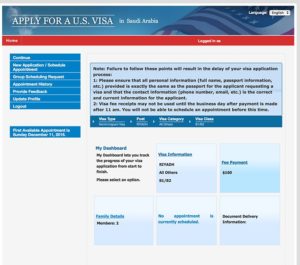A screenshot depicting a webpage designed for U.S. visa applications. The webpage features a vibrant, patriotically themed layout dominated by red, white, and blue colors. At the top, a blue banner with a semi-transparent U.S. flag on the right sets a formal tone. Below, a red banner spans the width of the page, creating a striking contrast against the remaining elements.

Beneath these banners, the page is divided into sections. The light blue clickable categories appear to organize various aspects of the visa application process, each providing detailed information. To the right of these categories, a column contains concise instructions, although the text is not fully legible in the screenshot.

Further down, a grid of six boxes offers additional categories or steps for exploring visa information and applications. The background is predominantly white, enhancing readability and emphasizing important details. A search bar located in the top right corner adds functionality, allowing users to quickly find specific information. The overall design reflects official U.S. thematic elements, promoting a sense of formality and reliability.